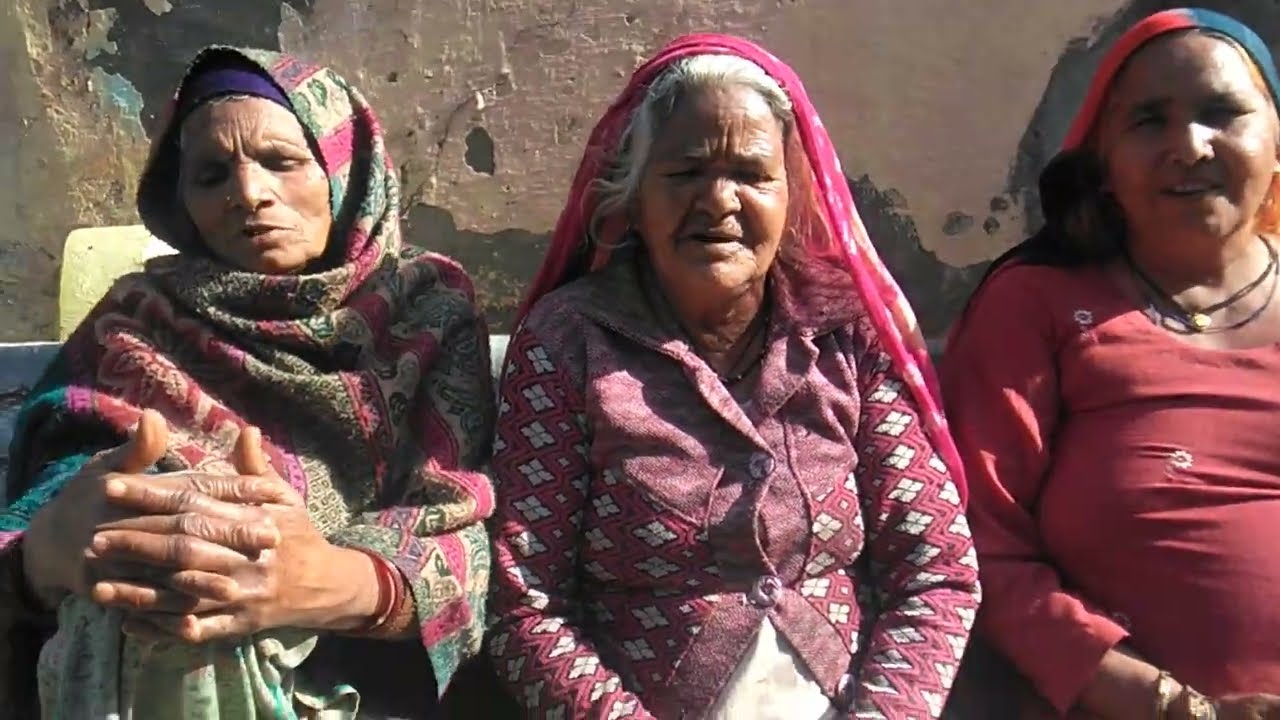This photograph showcases three older women seated side by side on a bench, basking in the outdoor sunlight. The background features an old, weathered concrete wall with chipping paint in shades of brown, gray, and light pink. Each woman wears distinct traditional headdresses, hinting at their indigenous heritage.

On the far left is an elderly woman, clad in a vibrant ensemble. She wears a purple headband, a poncho in shades of pink and gray, and a green dress. Her hands, resting on her knee, are notably wrinkled, suggesting her advanced age. Her shawl appears to be knitted with colorful patterns.

The woman in the middle, possibly the eldest, is donned in a pink shawl over her gray hair. She wears a pink sweater adorned with white floral patterns. Her eyes are closed, evoking a serene, almost prayerful demeanor. Her shawl suggests a handcrafted, possibly local origin.

The woman on the far right, appearing slightly younger than the others, has a fuller figure and sun-kissed brown skin. She sports a red shirt with floral designs, complemented by a red and blue headdress. Around her neck hangs a black necklace with a pendant. Her brown hair peeks out from under the scarf.

Together, these women create a vivid tableau of age, tradition, and cultural richness against the backdrop of a rustic, sunlit setting.